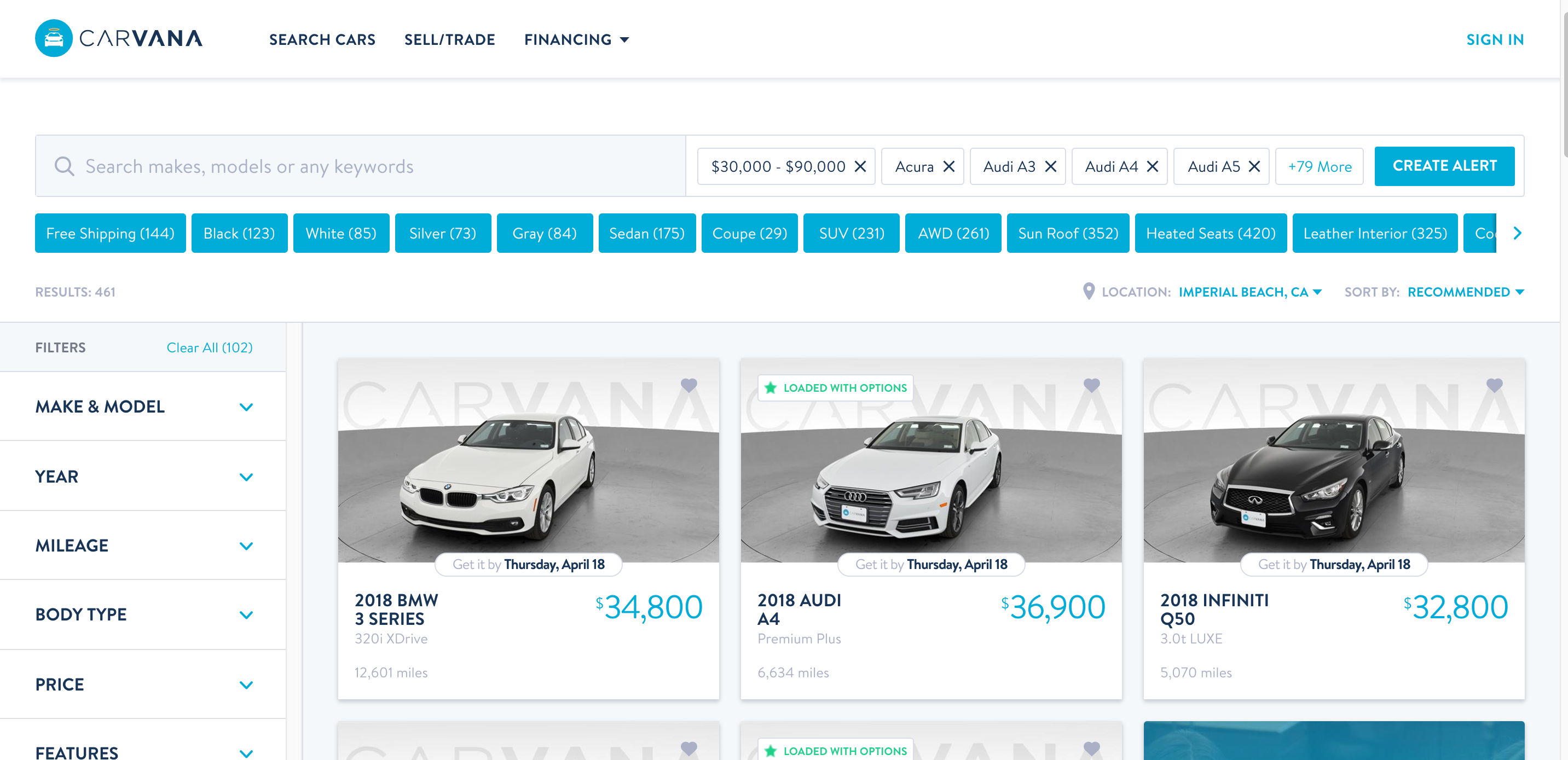The image showcases the Carvana website interface, set against a predominantly white backdrop, with black text and blue square icons highlighting different features. Centered at the top is a search bar, accompanied by a filter for price range, set between $30,000 to $90,000 in this instance. The user is interested in vehicles such as an Acura, Audi A3, Audi A4, and Audi AS, among 79 other options. Additionally, there is the functionality to create an alert for new listings. 

In the top right corner, there is a "Sign In" button also highlighted in blue. Notably highlighted features include free shipping, color options (black, white, silver, gray), and vehicle types such as sedan, coupe, and SUV. Further customization options are available for features like sunroofs, heated seats, and leather interiors, with specific filters tailored for Audi and BMW series showing the number of relevant cars.

On the left-hand side, a comprehensive filter panel allows users to refine their search by criteria including make and model, year, mileage, body type, price, and features, with an option to "Clear All" filters. Currently, there are 461 car listings that match the search criteria.

Three specific car listings are featured in the image:
1. A 2018 BMW 3 Series, priced at $34,800, is showcased in white against a showroom backdrop. This listing is from Thursday, April 18th.
2. A 2018 Audi A4, priced at $36,900, also in white, is highlighted for its extensive feature set. This car is likewise listed on Thursday, April 18th.
3. A 2018 Infiniti Q50, priced at $32,800, is presented in black, displayed on a similar showroom floor, and dated Thursday, April 18th.

The Carvana watermark is subtly present in the background of each vehicle listing, signifying the platform's branding.